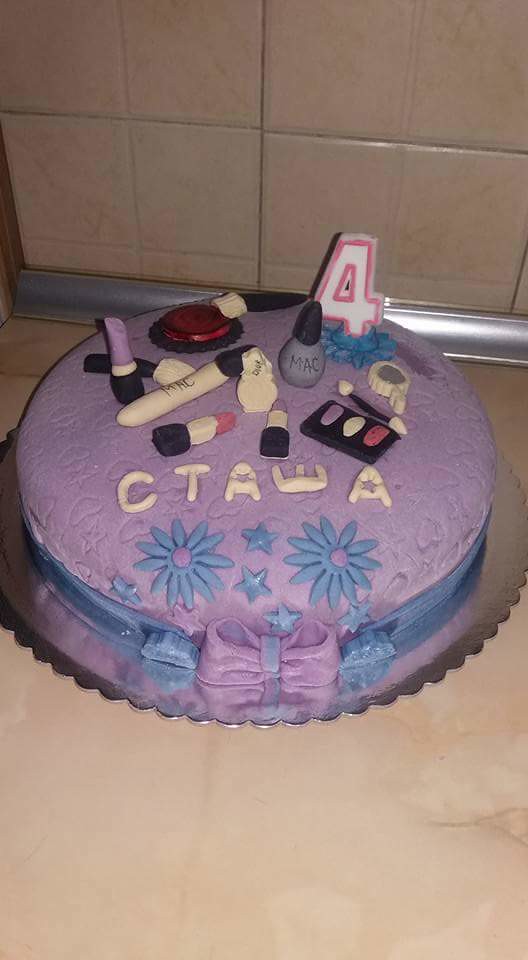This photograph captures a meticulously decorated birthday cake placed on a silver scalloped platter, which sits atop a tan granite countertop with a matching tan tile backsplash. The cake has a light purple quilt-like texture and features a striking array of edible decorations. Circling the bottom is a blue fondant ribbon with a purple bow in the front, flanked by two blue stars on either side. Above the ribbon, two blue daisies with purple centers are positioned to the left and right, with three more blue stars above and between them.

Prominently displayed in white lettering are the letters "CTAWA," positioned centrally just above the floral decorations. The cake’s top is festooned with various fondant-crafted makeup items, symbolizing a makeup kit. These items include tubes of purple and pink lipstick, a palette of red, white, and purple eyeshadow with an applicator, gray nail polish, blush with a brush, and a MAC-labeled bottle, indicating the popular makeup brand.

Crowning this elaborate design is an unlit number "4" candle outlined in pink, resting in the center of a flower, suggesting it's for a fourth birthday. The overall aesthetic fits a celebratory theme ideal for a makeup enthusiast, possibly a young girl.